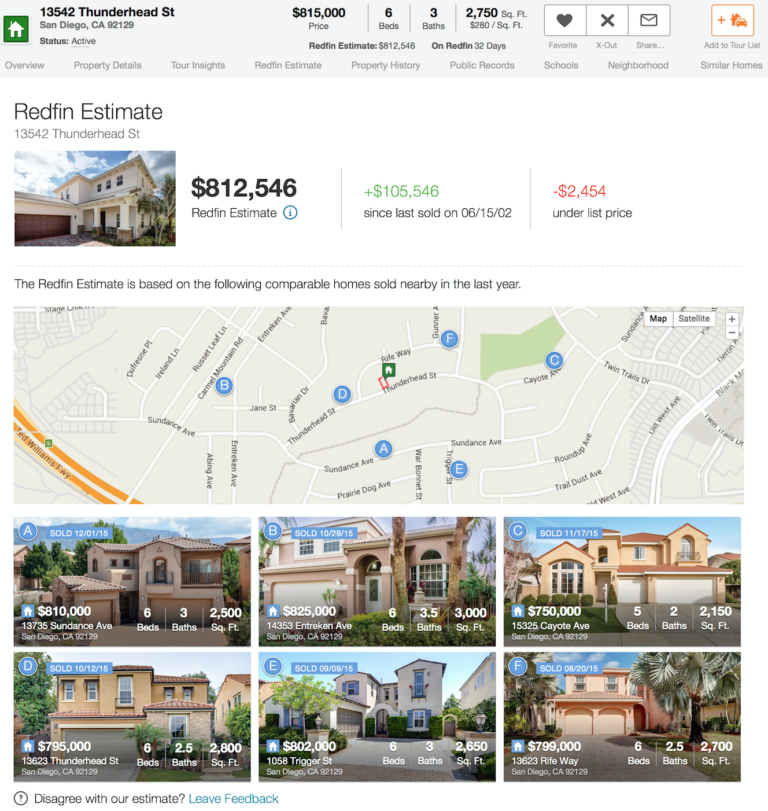This image features a detailed real estate listing on a white background. At the top, there's a blue box with listing information, and in the left corner, there's a small green box marked "House." The property is identified as 13542 Thunderhead Street, San Diego, California, 92129, with a status of "Active."

In the center, the price is prominently displayed as $815,000. Below that, it lists six bedrooms, three bathrooms, and a total area of 2,750 square feet. Accompanying this information are three icons: a heart, an X, and an envelope.

Further down, there’s a red plus mark box, a small red vehicle icon, and a house icon, indicating various features and amenities. Tabs for "Overview," "Property Details," "Tour Insights," "Rough Estimate," "Property History," "Public Records," "Schools," "Neighborhood," and "Similar Homes" are available for a thorough exploration of the property.

Next, a large white box details the Redfin estimate for 13542 Thunderhead, which is $812,546. It notes that this estimate reflects a $105,546 increase since the last sale on June 15, 2002, and is $2,454 below the current list price. The Redfin estimate is based on nearby comparable homes sold in the past year, with a small map showing the locations of several properties.

At the bottom, there are six high-quality images of beautiful nearby homes, listed with their respective prices: $810,000, $825,750, $795,000, $802,000, and $799,000.